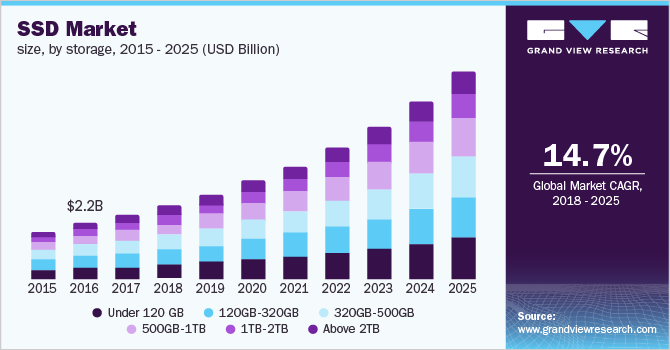The image is a detailed bar chart with a gray background, where the right side features a black section running from top to bottom. The caption on the very top left corner reads "SSD Market Size by Storage 2015 to 2025, USD Billion." The chart includes bars for each year from 2015 to 2025, and each bar consists of multiple colors representing different storage capacities. 

A table at the bottom indicates the color codes:
- Black: under 120 gigabytes
- Blue: 120 gigabytes to 320 gigabytes
- Teal: 320 gigabytes to 500 gigabytes
- Purple: 500 gigabytes to 1 terabyte
- Dark Purple: 1 terabyte to 2 terabytes
- Black: above 2 terabytes

Each bar increases in height from 2015 to 2025, showcasing graduall growth in SSD market size. For instance, the bar for 2016 is marked with 2.2 billion USD, while the tallest bar represents 2025.

To the right, there's a vertical banner with a purple and blue background. It reads "CVC Grandview Research," indicates a 14.7% global market CAGR from 2018 to 2025, and is sourced from www.grandviewresearch.com.